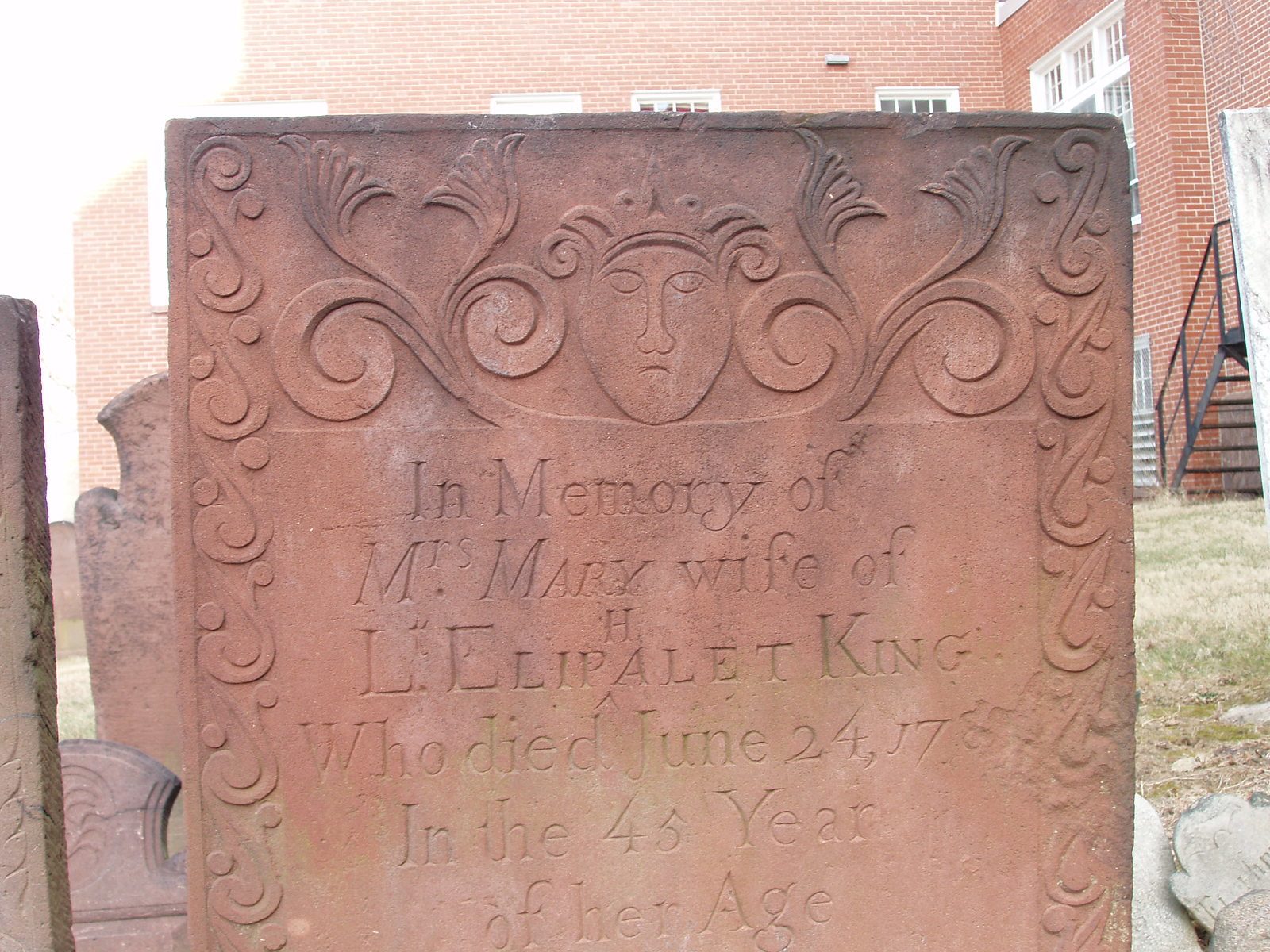The image is a detailed photograph of a rectangular, carved gravestone made from a red-brown type of stone. The stone features ornate etchings with curved lines along the sides and a stylized carving at the top depicting a person's head adorned with a crown. Inscribed on the gravestone is the text: "In memory of Mrs. Mary, wife of H. Eliphallet King, who died June 24th, 1780 in the 45th year of her age." The gravestone is set in a graveyard, with multiple other graves visible to the left. In the background, there's a red brick building with white windows, black metal staircases, and a clear sky, with grass covering the ground around the graves.